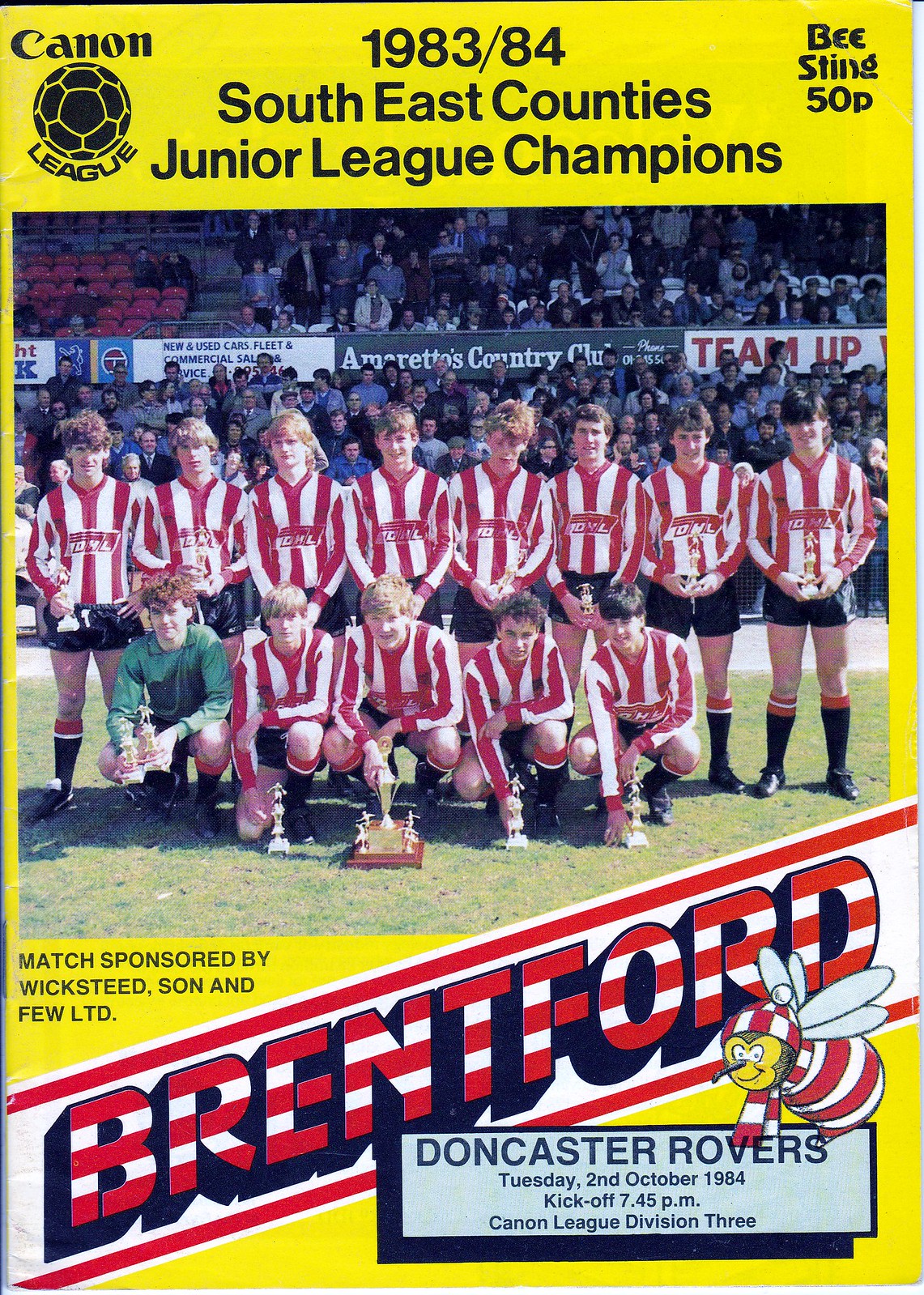The cover of the booklet is vibrant with a bright yellow background, prominently featuring a saturated color photograph of a soccer team. The team, likely an under-17 squad, is arranged in two rows, with the front row kneeling and the back row standing, all dressed in white and red vertically striped jerseys. Positioned on a lush green soccer field, they are backed by a stadium filled with spectators, adding a lively ambiance to the scene. At the center top of the cover, "Canon League" is displayed alongside a black soccer ball logo, indicative of the Canon camera brand, with "1983-84 Southeast Counties Junior League Championship" boldly marking the significance of the event.

In the corner of the upper right-hand section, the price "D. Sting, 50 pence" is mentioned. Dominating the bottom of the cover, large red and white striped text spells out "Brentford" beneath which details such as "Match sponsored by Wick’s Steed Sun and Few Limited" are provided. Notable is an advertisement for the Doncaster Rovers match on Tuesday, 2nd of October, 1984, with a kickoff time at 7:45 p.m., reinforcing the Canon League Division III context. A distinct logo resembling a bee, dressed in white and red stripes, is also showcased in the lower right side, adding an emblematic touch to the detailed, nostalgic cover.